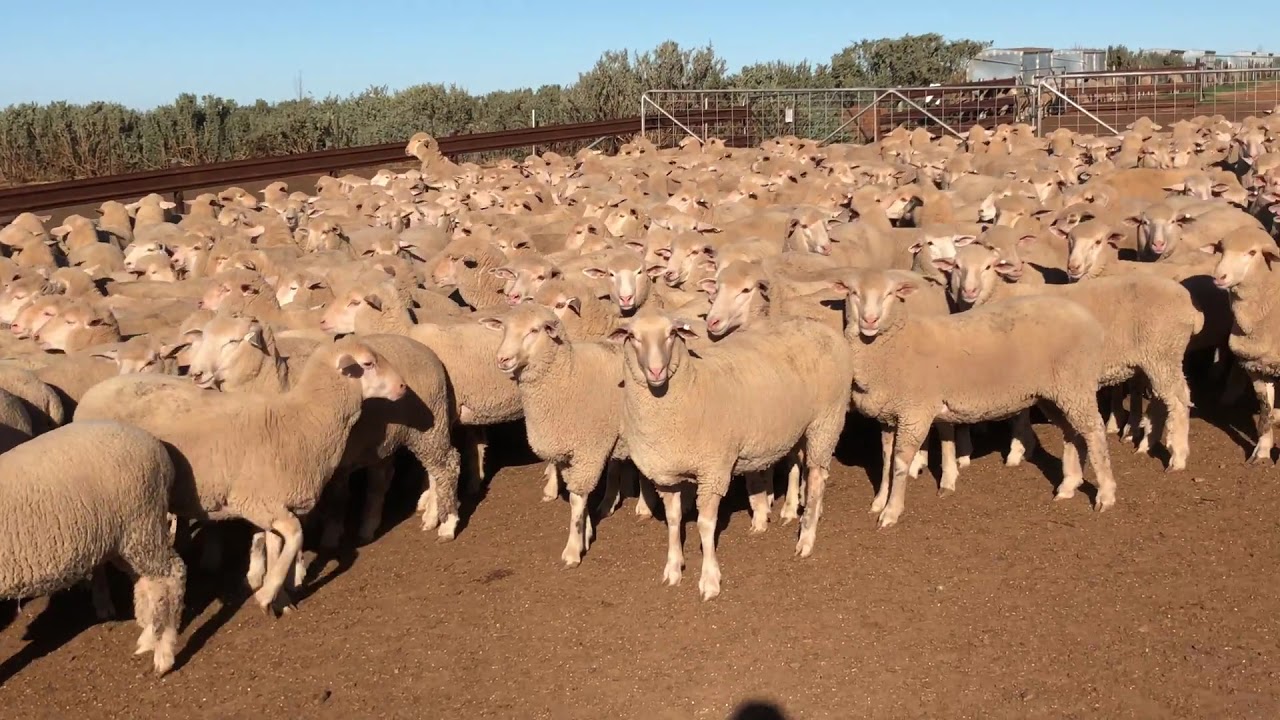In this outdoor photograph taken on a sunny day, a large flock of recently sheared sheep, each with a tag on their ear, is gathered in an enclosed area with reddish dirt flooring. The enclosure is bordered by a brown metal gate that can be partially seen. Most of the sheep are facing left, seemingly looking directly into the camera, while one sheep on the left stands facing the opposite direction. In the background, a couple of people stand near a silver gate, with a tree-lined horizon and a clear blue sky above. A wire fencing gate can be observed, with farm outbuildings further off in the distance. The lush green trees contrast with the vivid blue sky, adding a picturesque backdrop to the scene. At the very lower edge of the photograph, near the right center, the shadow of the person taking the photograph is faintly visible.